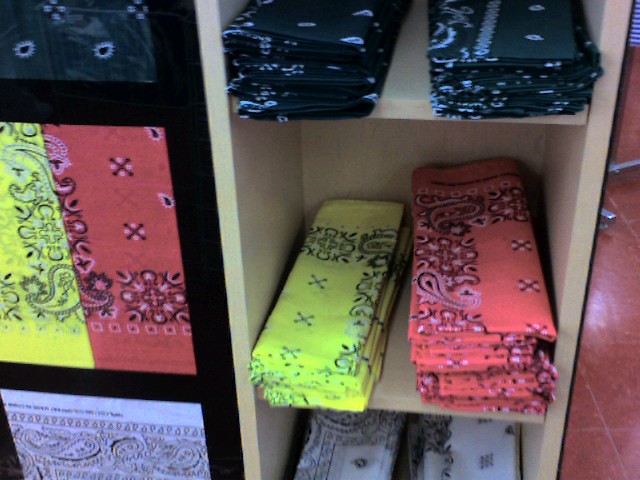This color photograph captures a detailed display of bandanas in a store. Situated in a cubby-like case with three vertical shelves, each compartment features neatly folded bandanas. The top shelf showcases bandanas with a dark fabric, possibly black or dark green, adorned with a white paisley design. The middle shelf prominently displays a striking highlighter yellow bandana, almost fluorescent green, with a black and white paisley pattern. This shelf also holds a stack of bandanas in a vivid carmine red, similarly decorated with black and white paisley accents. The bottom shelf features bandanas of white fabric with detailed black paisley designs. Adjacent to this cubby arrangement, there are smaller square samples showing the full pattern of each bandana for better visibility. On the far right of the image, part of a red-tiled floor is visible, contributing to the overall store ambiance. The photograph has noticeable film grain and pixelation, and there are no people, writing, or animals present in the scene.